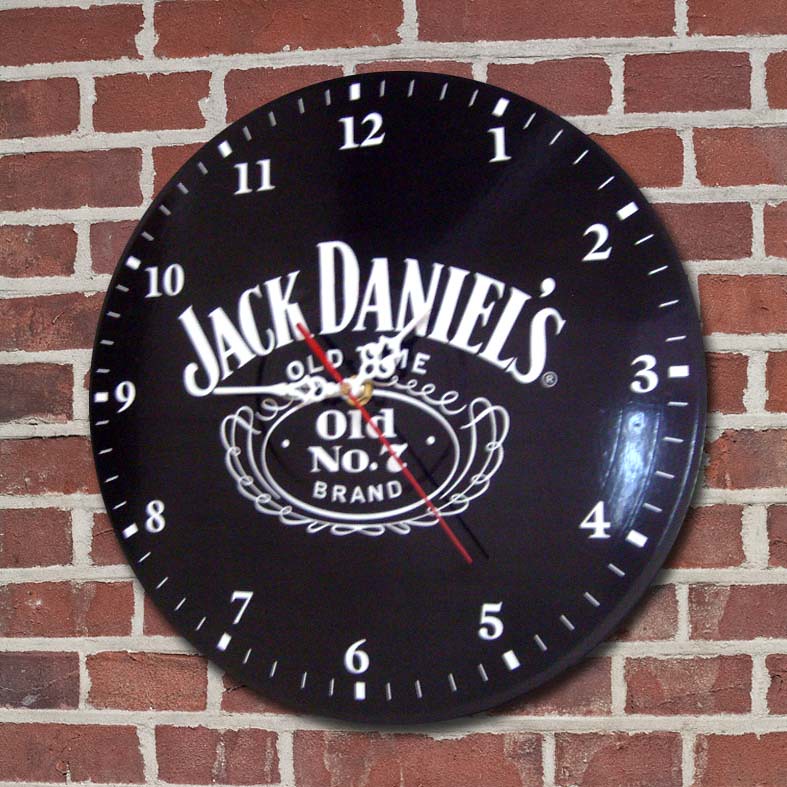The image depicts a large, circular black clock mounted on a weathered red brick wall with visible white grout and peeling plaster. The clock features bold white Arabic numerals from 1 to 12, with hash marks designating minutes and thicker rectangular ticks at each number. In the center, the face of the clock prominently displays the text "Jack Daniel's Old Time Old No. 7 Brand" in white lettering, with a medallion-like design surrounding the brand statement. The clock's hour and minute hands are intricately detailed with white scrollwork, while the thin, straight second hand is distinctively red. The time on the clock reads 1:45, with the second hand pointing to the 5.